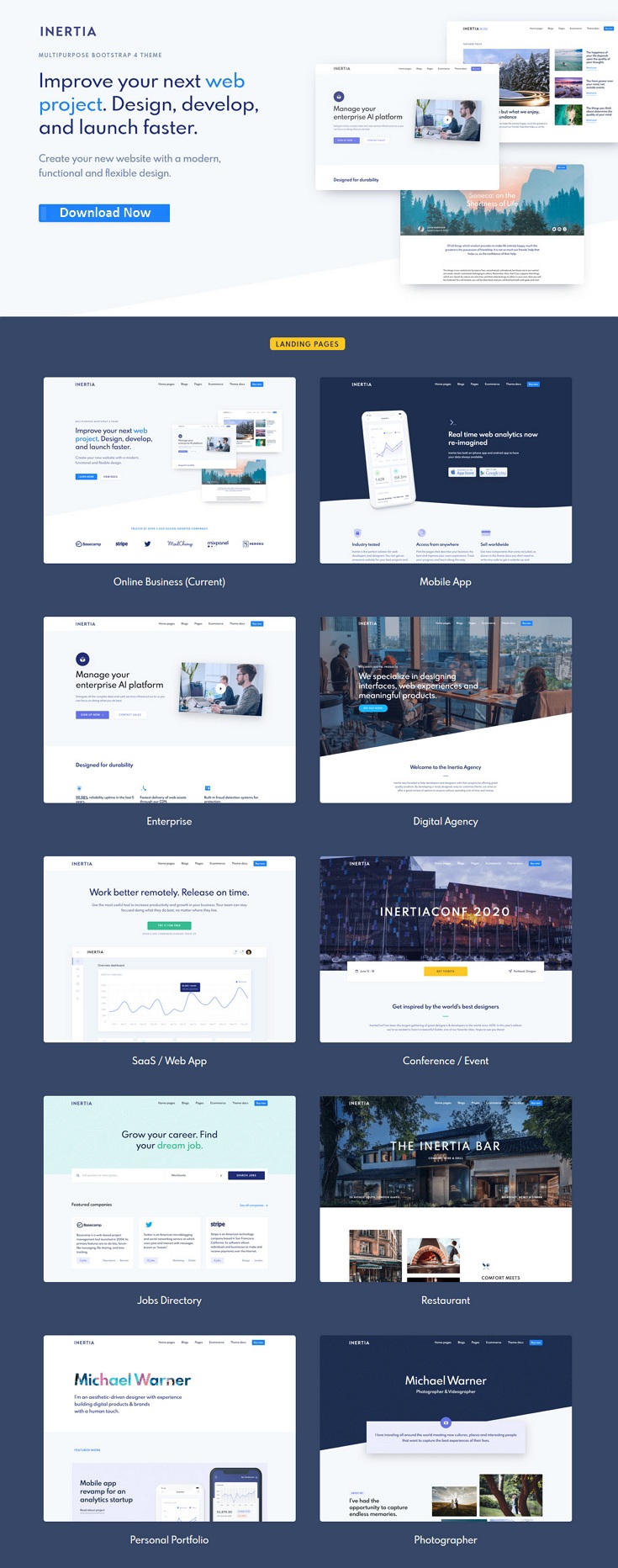This image depicts a screenshot from software presented in a portrait format, likely from a mobile device or tablet. The header of the software interface prominently displays the word "INERTIA" in uppercase letters. Below the header, a tagline reads, "Improve your next web project: design, develop, and launch faster," with "web project" highlighted in blue to draw attention. Directly beneath this tagline is a blue button with white text that reads, "Download Now."

To the far right, there are several small screenshots of the software itself. These include an image of people seated in what appears to be an office or conference room, and another screenshot featuring an illustrated landscape background. The images are rather small, making detailed observation difficult.

Further down, against a dark grey-blue background, there are 10 template options available for structuring the initial interface of a website, though the options are too tiny to be clearly visible. At the bottom, the name "Michael Warner" is mentioned, potentially signifying the company associated with the software.